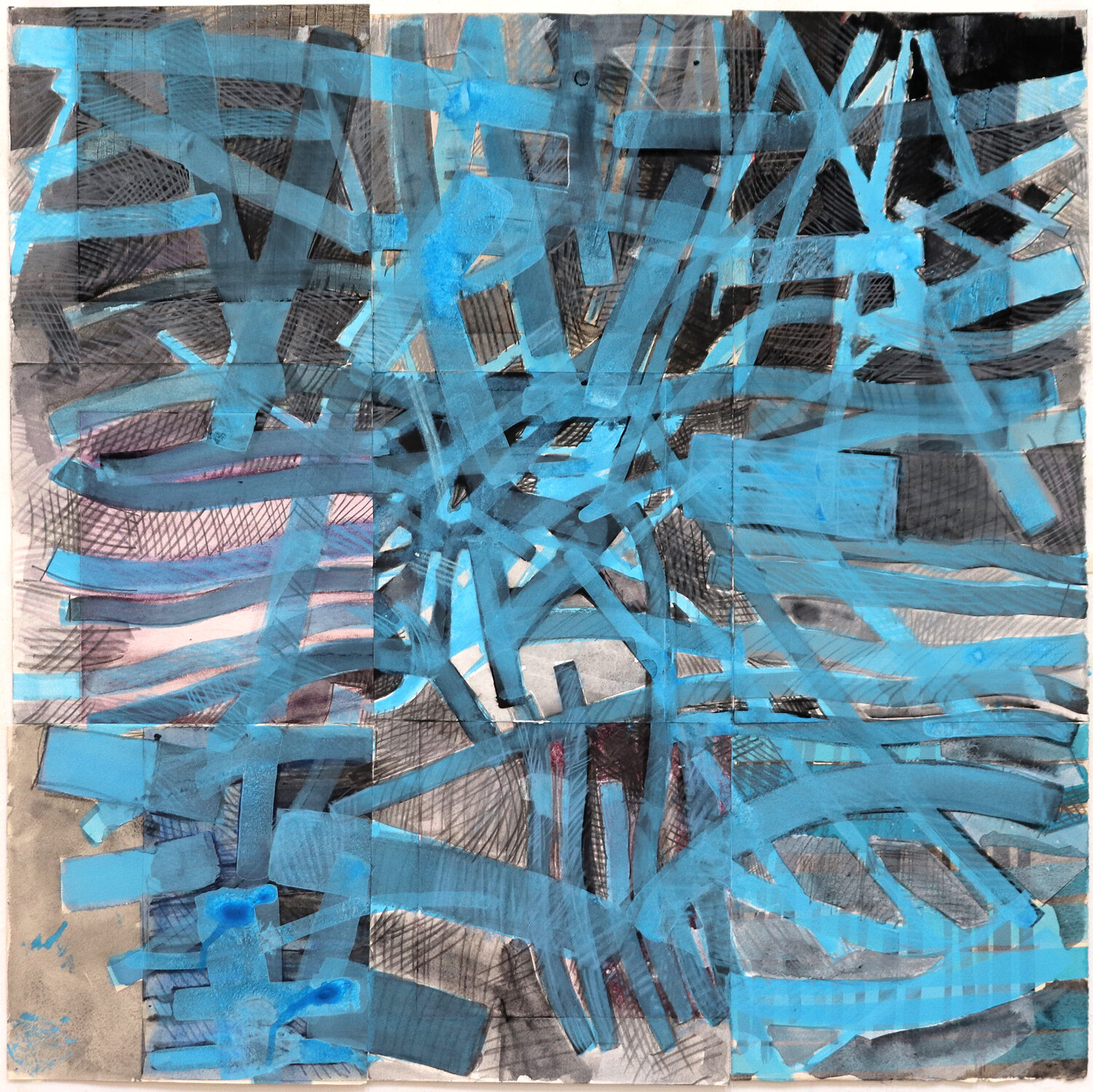This image features a square-format modern art piece titled "Reconvene" by Julie Shapiro. It is composed of three wooden planks or blocks arranged in a 3x3 grid. The background of the artwork showcases a cross-hatching design created with ink hash marks in black and gray tones. Overlaying this intricate backdrop are multiple intersecting lines and shapes rendered in aqua blue paint. These lines vary in thickness, direction, and pattern—some curved and some angular—extending across the image from left to right and from top to bottom. At the center of the composition, where several lines converge, a 3D effect is emphasized through dark shadowing, giving a sense of depth and complexity. The overall abstract design is a striking example of color painting art.